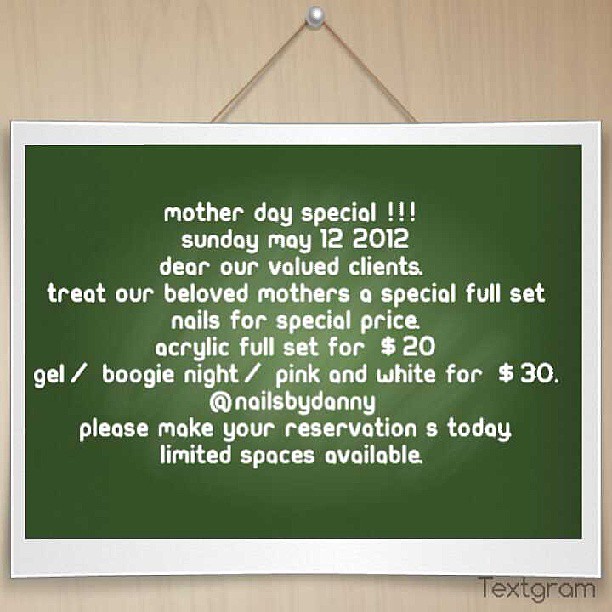The image is a colorful, cartoon-like clipart picture of a green chalkboard sign hanging by strings from a wooden panel. The chalkboard features a white font with the announcement: "Mother's Day Sale! Sunday, May 12, 2012." Addressing valued clients, the sign encourages them to treat beloved mothers to a special offer on nail treatments with details such as, "Acrylic Full Set for $20" and "Gel/Boogie Night/Pink and White for $30," with the disclaimer, "Please make your reservations today; limited spaces available." The services are provided by "Nails By Danny." The bottom right corner of the chalkboard has a watermark reading "Textgram." The text is entirely in lowercase with inconsistent punctuation, enhancing the quaint, homemade feel of the advertisement.